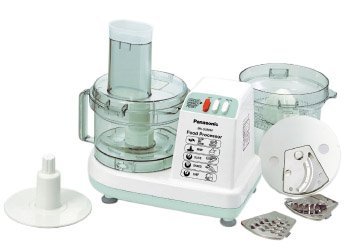The image showcases a small, Panasonic-branded food processor with a clear plastic container featuring a long feeder tube. The processor itself is predominantly white with light green accents. The front panel displays various settings in labeled rectangles, and there are three buttons—a red button followed by two white ones. The food processor is accompanied by multiple accessories, including a white chopper attachment, two different graters, a white disc shredder, and an additional bowl. Silver metal parts for cutting are visible, positioned on the right side of the machine. The main container with the feeder tube is attached to the food processor, while another bowl sits behind it. Additional lids and various blades are also arranged around the food processor. The overall setup is devoid of any background, focusing entirely on the product and its accessories.